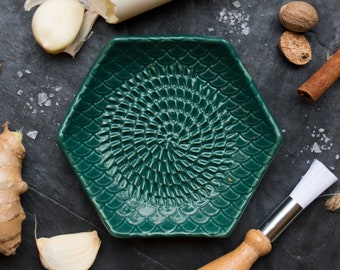This rectangular image, wider than it is tall, presents a detailed, professional photograph showcasing a culinary scene. Set against a gray background that resembles a slate or stone countertop, the scene features a distinctive hexagonal dish at its center. The dish, with its dark green, jade-like hue that lightens towards the bottom, features an intricate pattern transitioning from scale-like designs along the edges to a circular, flower-like motif in the center. The dish, empty and pristine, is surrounded by a variety of items including ginger, garlic, nutmeg, a walnut, and possibly some onions. There are traces of white residue that might be salt sprinkled around, adding texture to the scene. A cooking utensil can also be spotted among these items, contributing to the overall impression that this could be a meticulously arranged setup for an advertisement or social media post.